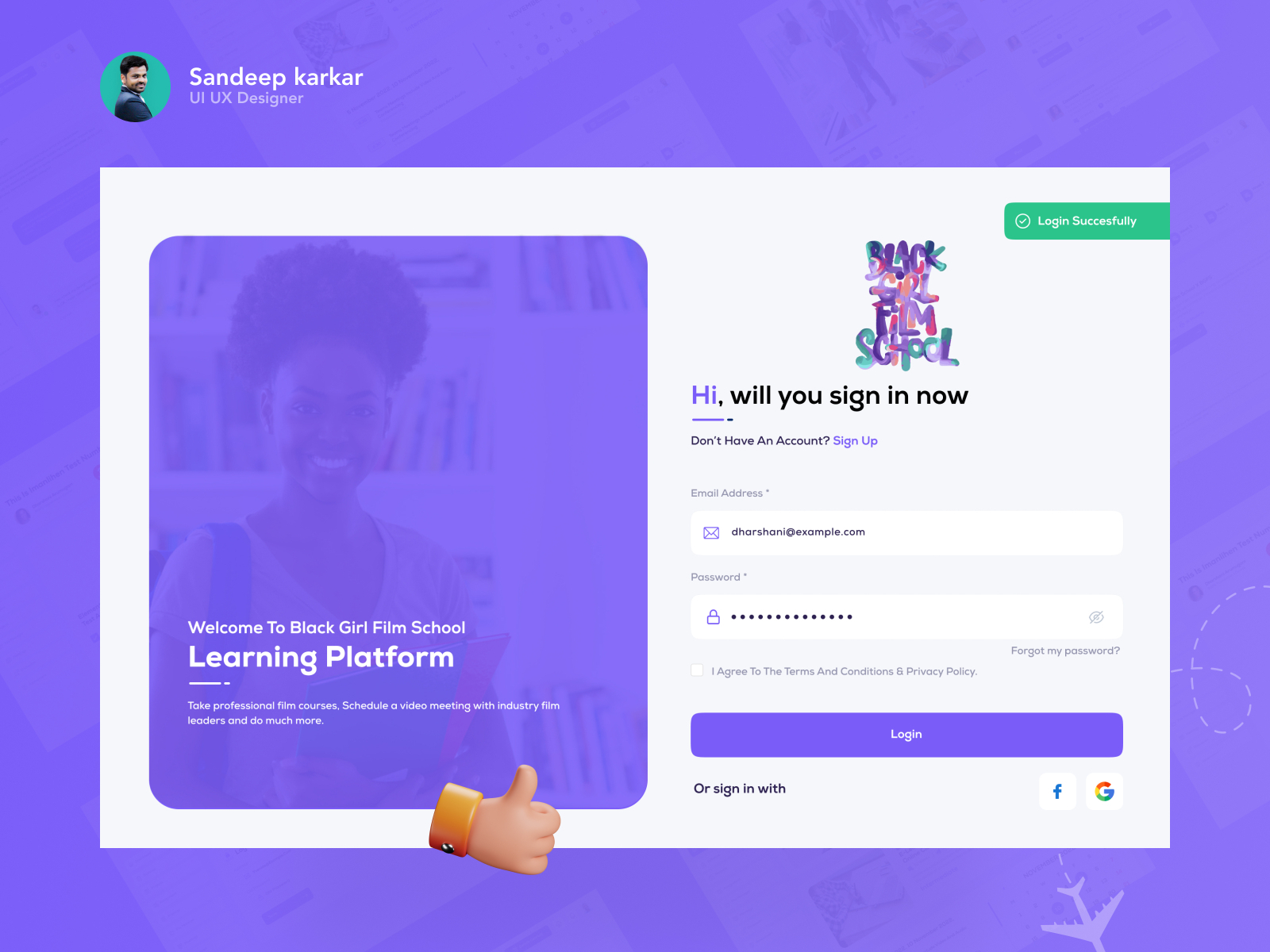The image is a detailed screenshot from a website. The background features a bright purple square. At the bottom of the image, there are graphics that include an airplane descending with a dotted line trailing behind it. The scene also includes cartoon-like characters, not actual people. In the top left corner, there is a green circle containing a stylized figure of a person turning their head over their right shoulder. The text beside the circle reads "Sandeep Karkar," spelled "S-A-N-D-E-E-P K-A-R-K-A-R," with the title "UI/UX Designer."

Beneath this section, there is a white square, which contains another smaller square of the same bright purple color as the background. This inset square shows a silhouette of a person’s face, artistically rendered with visible features. Accompanying it is the text: "Welcome to Black Girl Film School Learning Platform."

Further down, there is text prompting the user to sign in: "Hi, will you sign in now? Don’t have an account? Sign up." Below this, there are fields labeled for an email address and password, followed by a checkbox for agreeing to the terms and conditions and privacy policy. Finally, there is a "Log In" button.